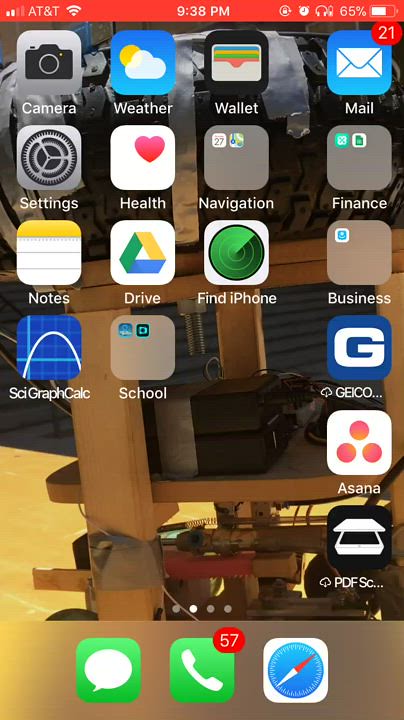This stylized poster depicts a vertical view of a tablet or iPhone screen, vividly showcasing various installed apps. At the very top, a narrow red bar prominently displays essential information. On the left, the provider "AT&T" is indicated, with excellent signal strength denoted by full bars. Centrally placed is the time reading "9:38 p.m." in white text. The right side of the bar includes symbols indicating connected headphones and a battery level at 65%.

The main screen features a structured layout of apps arranged into four columns and seven rows, with the top three rows filled entirely with four apps each. Progressing downward, the arrangement displays three apps in the fourth row, one in the fifth and sixth rows, and three in the seventh and final row. 

The icons represent a variety of applications, including Camera, Weather, Wallet, Mail (showing 21 unread messages), Settings, Health, Navigation, Finance, Notes, Drive, Find iPhone, Business, SciGraphCalc, School, Geico, Asana, and PDFSC. 

At the bottom, three distinct icons in green squares with rounded corners indicate key functions: a messaging bubble for Messenger, a phone icon with 57 missed calls, and a compass displaying a blue background with a red and white needle.